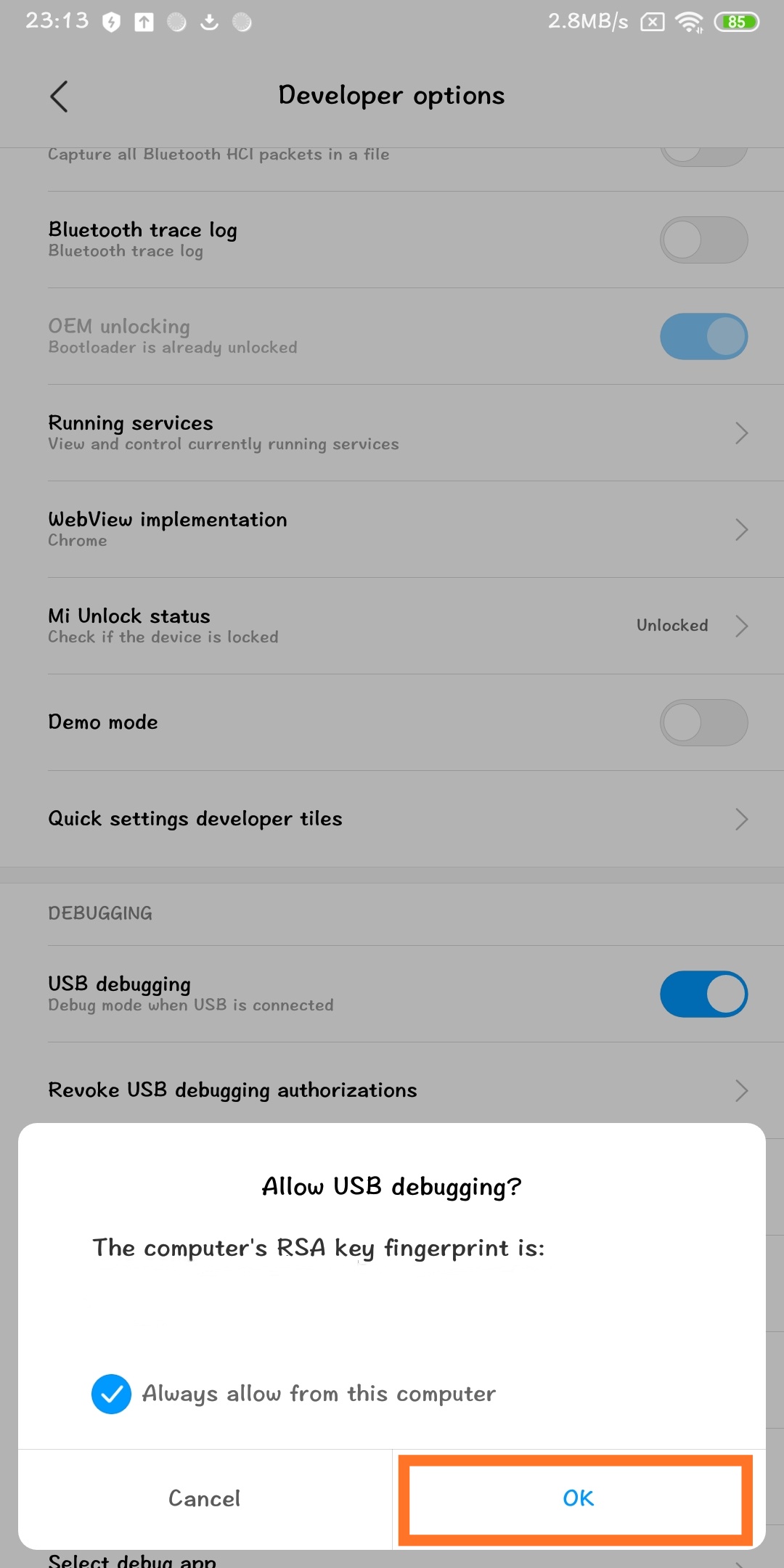A cell phone screenshot displaying various on-screen elements. The background, originally white, appears grayed out. The system font used is Comic Sans. 

The top bar shows the time as 23:30, with a shield icon, an upward arrow enclosed in a circle, and another circle icon. On the right side are the text "Why Europeans know what their speed they have to get all the time" at 2.8 MBs per second, and a notification indicating that no SIM card is installed. Wi-Fi is shown as fully connected, and the battery icon, green and partially charged, shows 85%.

A black arrow points left towards various developer options such as "Developer Options," "Running Services," "OEM Unlocking," "Web View of Information," "Demo Mode," and "Quick Settings and Developer Tiles." Another notable option, "USB Debugging," is turned on, which opens a pop-up window.

The pop-up window has a white background with the text: "While USB debugging, the computer's RSA key fingerprint is:" followed by an empty space. Below this is a blue checkmark next to the option "Always allow from this computer." At the bottom, there are two buttons: "Cancel," outlined in an orange rectangle, and "OK."

This detailed description covers all the visible elements in the screenshot.